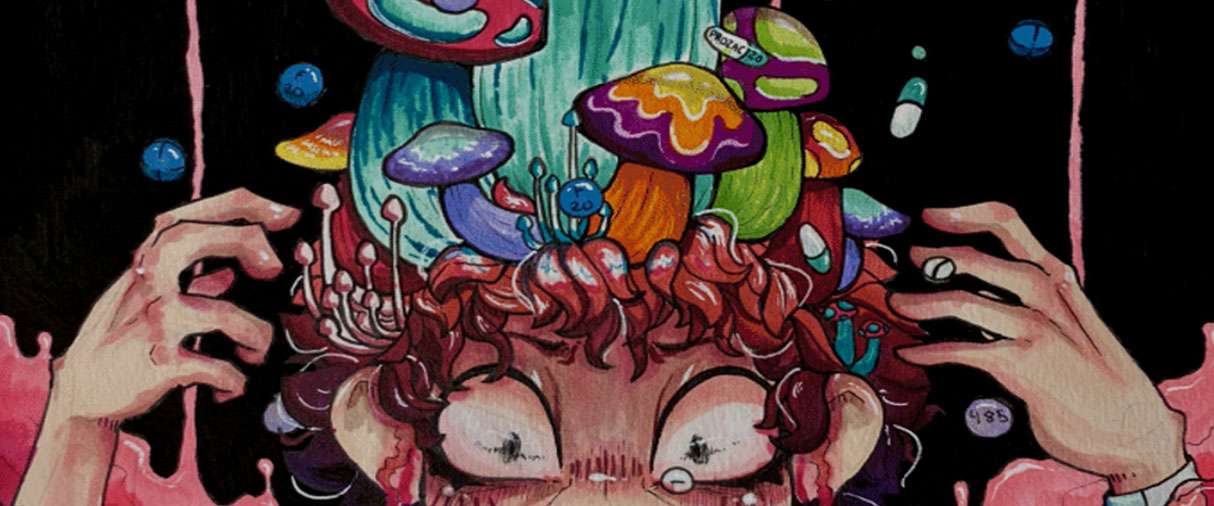This intricate and colorful drawing features the top of a person's head, seemingly exploding with vibrant hues and a fantastical array of mushrooms and fungi. The person, with distinctly reddish hair, has light-colored skin, suggesting a Caucasian ethnicity. The mushrooms sprouting from the scalp display a variety of colors: an orange-stemmed mushroom capped in purple, orange, and yellow; a blue-stemmed mushroom with a blue and white top; and a brown-stemmed mushroom on the right side with a brown and white cap. Among these, blue-colored circles add to the whimsical scene. 

In the upper part of the image, bubblegum-colored paint appears to be dripping and splashing downwards, enhancing the surreal aesthetic. Two hands extend from the left and right corners toward the head, their fingers poised as if about to grasp the fungi. This artistic depiction has a futuristic vibe, emphasized by the blue and white capsule floating in the black upper background and the marble-sized blue balls scattered above. The lower section of the background features pink wavy patterns originating from both corners, behind the hands. Additionally, the number "485" is subtly inscribed in white beneath the right hand, contributing a mysterious numeric element to the overall composition.